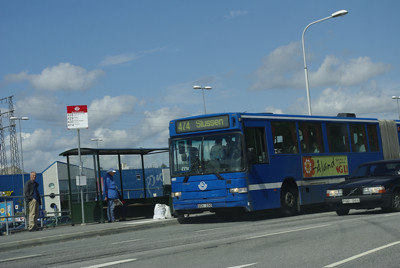In this detailed photograph, we see a deep blue articulated bus with an accordion joint, signaling its length, as it approaches a bus stop on a paved gray asphalt road. The bus carries an advertisement on its side, which features a yellowish green background with a red flower and black lettering, though the text is difficult to discern from this distance. The bus is identified as route 474 with the word "SUSSEN" displayed above the driver’s window. The driver and a passenger are faintly visible through the windshield.

Adjacent to the bus is a black Volvo with distinctive lights and a white European license plate, both seemingly moving side-by-side. The road is marked with white lines delineating different lanes, suggesting a four-lane road with two lanes in each direction.

The scene includes a bus stop with a glass or plexiglass shelter supported by brown bars, designed for waiting passengers. There are two people at the bus stop; one woman dressed in a long sleeve blue jacket and jeans, wearing a discreet cap, stands in the shelter, while a man in a black long sleeve jacket and khaki pants stands outside. Positioned between them is a tall pole bearing a red and white sign, likely indicating bus routes and schedules, with additional details that are not fully readable from the photo. The sky is a bright blue with wispy and puffy white clouds scattered across it, and overhead lighting fixtures are visible above the street.

In the background, several sheds and additional urban elements add to the depth of the scene, capturing a typical day in a seemingly European city.